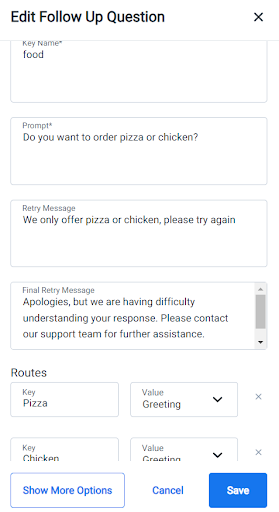This is a detailed screenshot of an interface titled "Edit Follow-Up Question," prominently located in the top left corner of the page. On the top right, there is an "X" button for closing the interface. Below the title, there are multiple fields for input, each clearly labeled.

The topmost field is labeled "Key Name" and is marked with an asterisk to indicate it is a required field. Beneath this label, the text "Food" is entered. The field immediately following is labeled "Prompt," also marked with an asterisk, with the text "Do you want to order a pizza or chicken?" entered beneath it.

The next field is labeled "Retry Message," containing the text, "We only offer pizza or chicken. Please try again." Following this, there is a section labeled "Final Retry Message," which contains the text, "Apologies, but we're having difficulty understanding your response. Please contact our support team for further assistance."

Below these sections is an area labeled "Routes," which has rows consisting of two fields each. The first row contains a "Key" field with the value "Pizza," and its corresponding "Value" field is set to a dropdown option labeled "Greetings." The second row similarly contains a "Key" field with the value "Chicken," and its corresponding "Value" field is also set to a dropdown option labeled "Greetings."